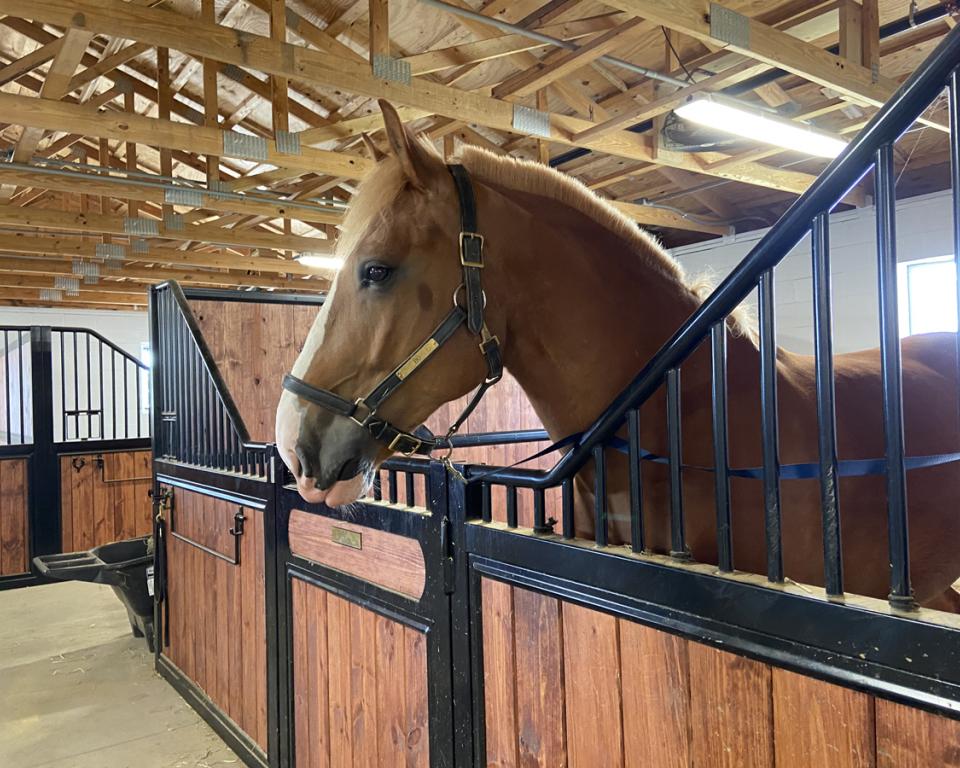The image showcases a well-groomed light brown horse with a freshly trimmed mane and a distinctive white stripe running from between its eyes to the tip of its nose. The horse, which has a black bridle, is standing attentively within a meticulously maintained, open-ceiling barn. Inside its wooden stall, reinforced with black metal bars, the horse appears eager and alert, its ears pointed forward. This intricately constructed stall features a gate with an unreadable plaque, possibly indicating the horse's name. In the background, a hay barrel can be seen, suggesting the barn's functional purpose. Underneath the metal bars of the stall is a rich mahogany-colored wood, hinting at an environment designed for showcasing well-cared-for horses. The scene is bathed in fluorescent light illuminating the horse and its surroundings, highlighting the barn's new, polished condition.